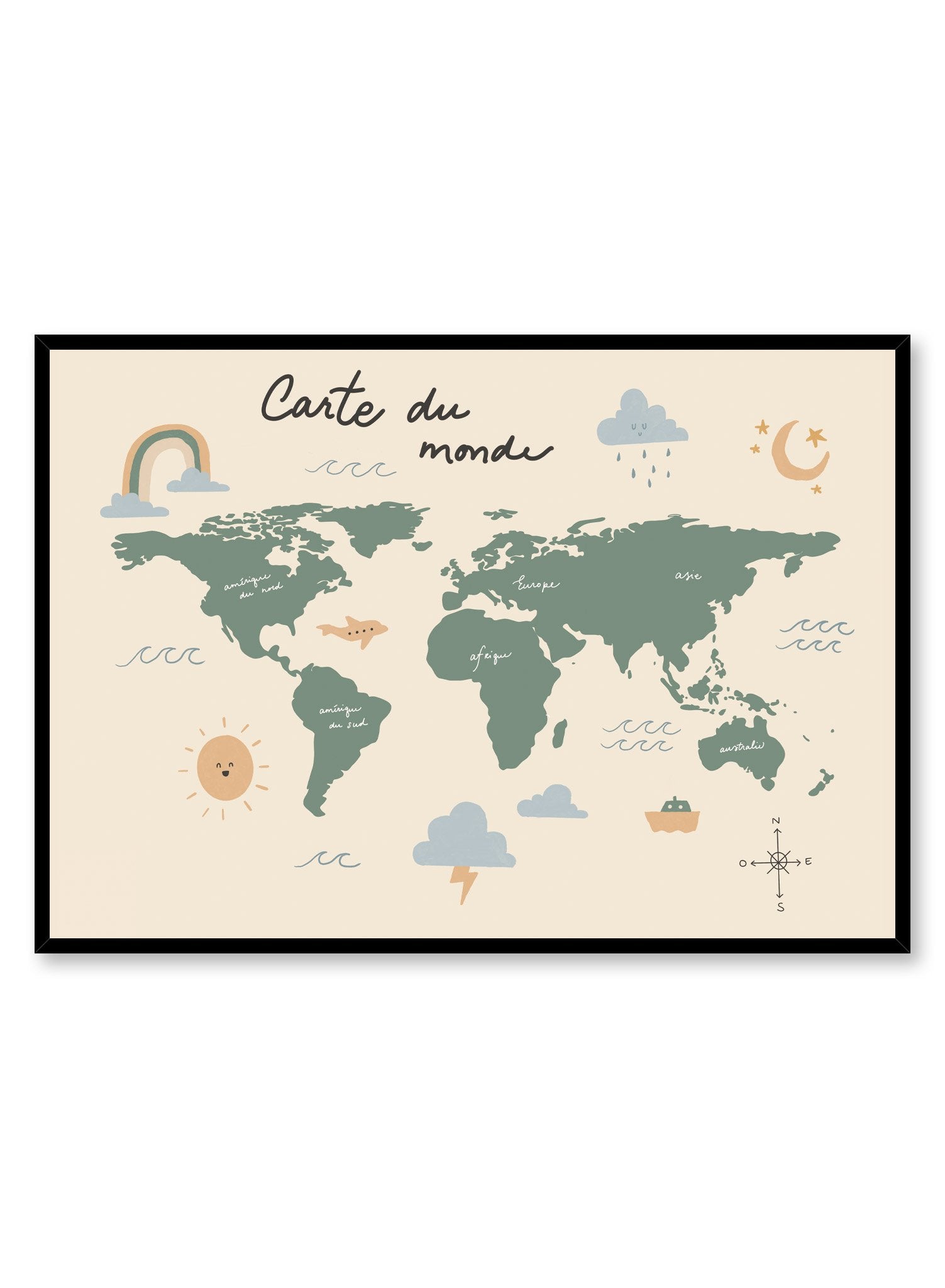This striking image, titled "Carte de Monde," presents a contemporary and detailed graphic drawing of the world map. Framed in black against a white background, the map showcases the world's continents in vibrant green, with their names elegantly inscribed in white script. The continents span from the Americas on the left to Asia and Australia on the right, though neither the Arctic nor Antarctic regions are depicted.

The map is surrounded by charming, cartoonish illustrations contributing to a weather and nature theme. A cheerful sun with a smiley face, a crescent moon, and a whimsical rain cloud with a face add a playful touch to the piece. Additional weather elements like a rainbow, thunderbolt, and raindrops are distributed around the map. In the lower sections, a small fishing boat navigates the waters below Australia, while a compass in the lower right ensures directional accuracy.

Completing the composition are delightful images of a whale and various weather-related icons, enhancing the map's vibrant storytelling. The title, "Carte de Monde," is handwritten at the top, indicating that the map is labeled in French. This detailed and colorful depiction makes the map both an educational tool and a piece of art.